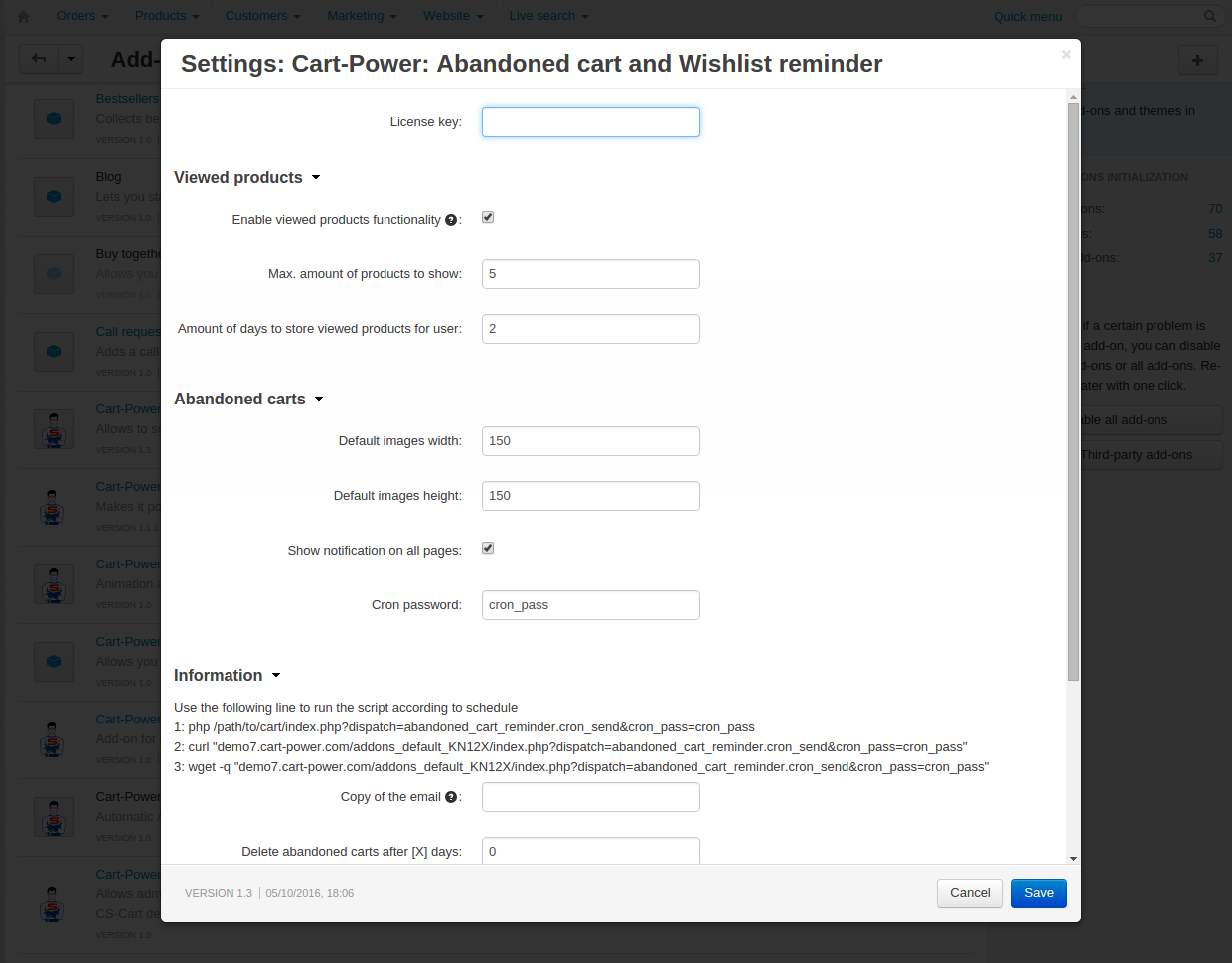The image displays a user interface of a webpage surfaced within another larger, darker webpage. The primary focus is a popup window with a white background containing settings options and various input fields. Behind this popup, the larger black page is visible but blurry, displaying indistinct icons and text. The settings window is clearly legible and includes multiple sections:

- **Main Options**: 
  - "Settings"
  - "Cart Power"
  - "Abandoned Cart"
  - "Wishlist Reminder"

Additional settings options:
- **License Key**: A text box for entering the license key.
- **Viewed Products**: A checkbox labeled "Enabled Viewed Products and Functionality" which is checked, indicating the feature is active.
  - **Max Amount of Products to Show**: Set to 5.
  - **Amount of Days to Store Viewed Products for User**: Set to 2 days.
- **Abandoned Carts**:
  - **Default Width**: Set to 150 pixels.
  - **Default Height**: Set to 150 pixels.
  - **Show Notification on All Pages**: This checkbox is checked.

Additional configurations:
- **Cron Settings**:
  - **Cron Password**: "cron_pass" is displayed in an input box.

The bottom right of the popup window features two buttons:
- **Cancel**: Option to discard changes.
- **Save**: Highlighted in blue, indicating it is the primary action.

Below these buttons, instructional text provides information:
- "Use the following line to run the script according to schedule" followed by a step-by-step guide.